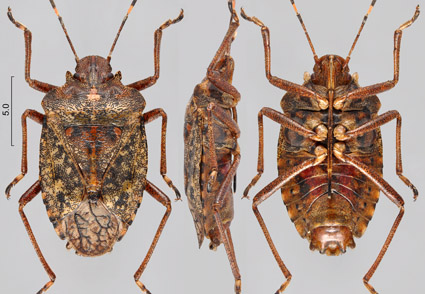The image features three detailed photographs of a beetle, each taken from a different angle: an overhead view on the left, a side profile in the center, and an underside view on the right. A vertical black line labeled "5.0" on the left provides a scale for measuring the beetle's size. The beetle is predominantly brown with patches that appear red and purple, and its legs are notably long and intricate. In the overhead view, the light brown antennae, adorned with yellow stripes, are prominently extended, while the legs exhibit distinct upward and outward patterns. The side profile captures the beetle’s legs aligned in a straight line, emphasizing the form and structure. The underside view reveals bright orange spots where the legs attach to the body. The beetle’s body features a mix of black and yellow spots with touches of brown and red in the middle. The background of the entire image is a light gray, providing a stark contrast that highlights the beetle’s vibrant details. The lighting is bright and even, ensuring all features are clearly visible.